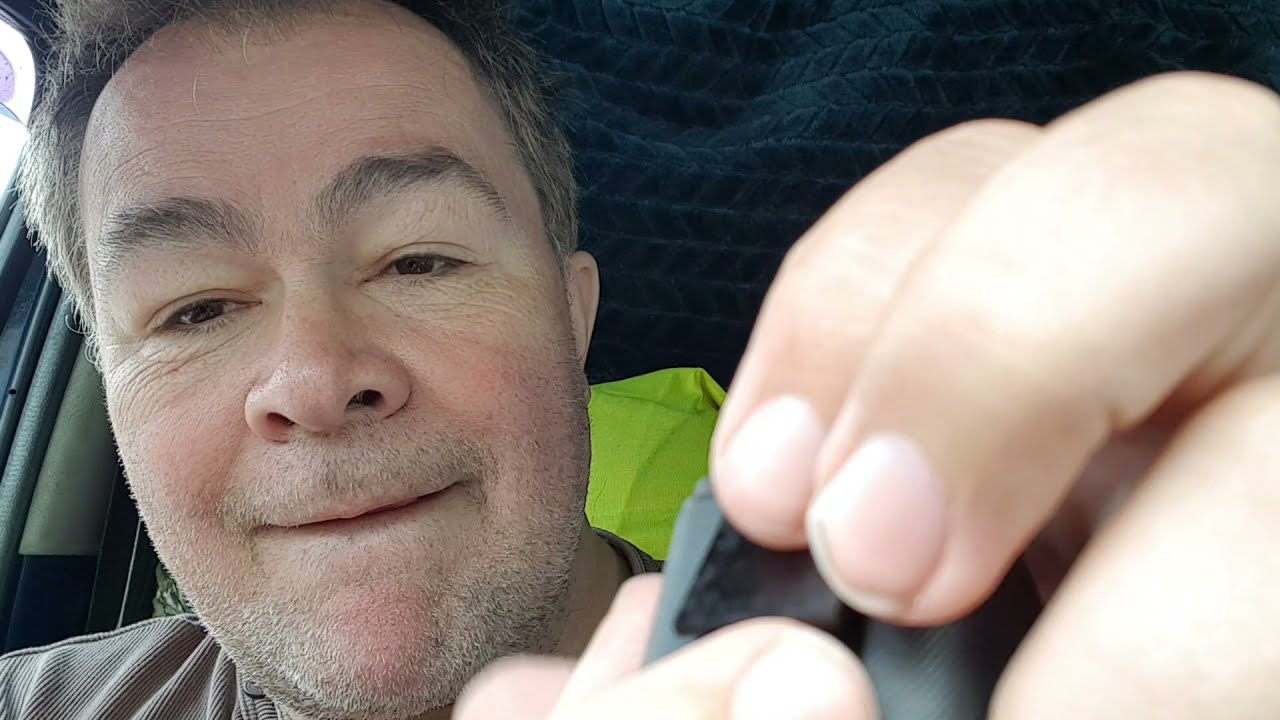This horizontal rectangular close-up image shows an older man, likely in his late 40s to early 60s, inside a vehicle. Positioned on the left side of the frame, his head is slightly tilted, revealing his short salt-and-pepper hair and raised eyebrows. His mouth is slightly open with his lips curled under in a slight grin, accentuating the stubble around his mustache and beard area, which is a mix of brown and gray. On the far left, part of a window and the seatbelt area are visible, indicating he is in the driver's seat.

In the background, above his head, hangs a black fabric with a rectangular pattern, possibly a blanket, adding texture to the scene. His right shoulder is just visible in the lower left corner, clad in a textured brown, button-down shirt. On the right side of the image, a somewhat blurred close-up of his hand holds a small gray package with a black tab in the middle, suggesting it might be something he is about to open. The overall setting hints that it is daytime and the man is inside his parked car. The image features shades of tan, gray, black, brown, light green, dark green, and silver.